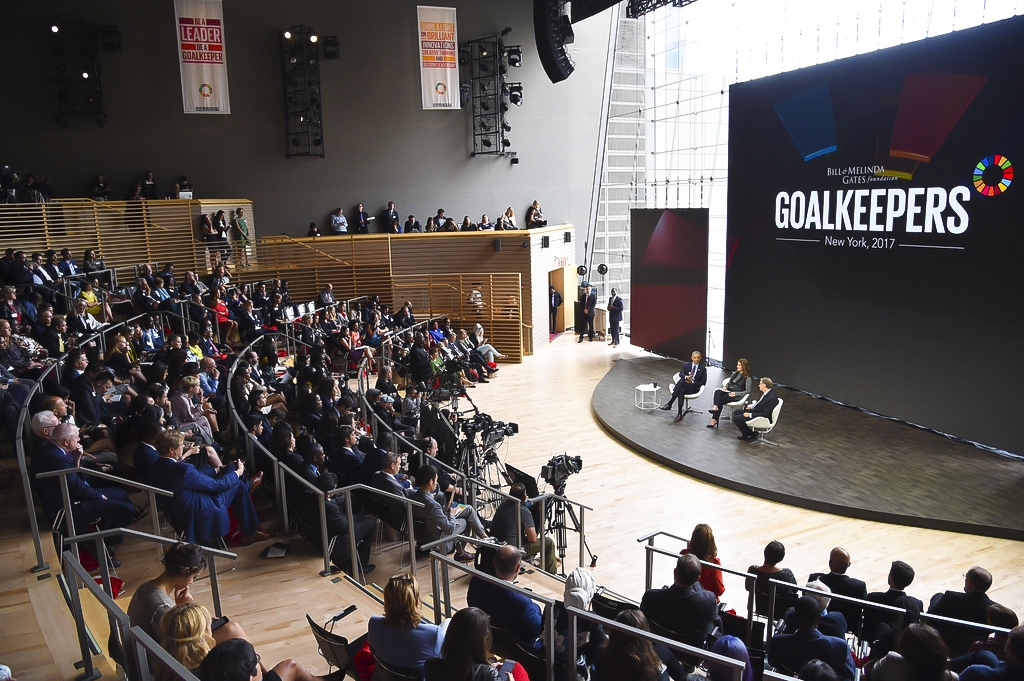The image depicts a realistic, slightly horizontally oriented photograph of an auditorium or stadium, likely set up for a large-scale lecture that accommodates several hundred people. The right side of the image prominently features a large backdrop sign reading "Bill and Melinda Gates Foundation Goalkeepers New York 2017," with a circular emblem depicting a multi-colored design. This sign is part of the backdrop and is set against a large window.

On the lower part of the auditorium, situated on a slightly elevated, curved brown stage that appears to be only a few inches off the ground, three individuals are seated. They are presumed to be Bill and Melinda Gates and another man who might be a moderator or interviewer. All three are dressed in business attire; the men in suits and the woman in professional dress. They sit on white chairs, accompanied by a small white table next to the man on the left. 

In front of this trio, the audience is arranged in a semi-circular fashion, seated in a tiered, bleacher-style setup that somewhat resembles a mini arena or a lecture hall. The attendees, dressed in business casual attire, appear to be attentive adults, possibly journalists or professionals, who are focused on the stage. The event is evidently formal, as suggested by the presence of video cameras and lighting equipment, indicating that the session is being recorded.

The back wall of the auditorium features some signs and lighting fixtures, though the details on these signs are not fully legible from the provided viewpoints. Security personnel are noted to be standing off to one side, ensuring the smooth running of the event. Overall, the photograph captures a business-oriented event where Bill and Melinda Gates are presumably discussing philanthropic goals or initiatives.